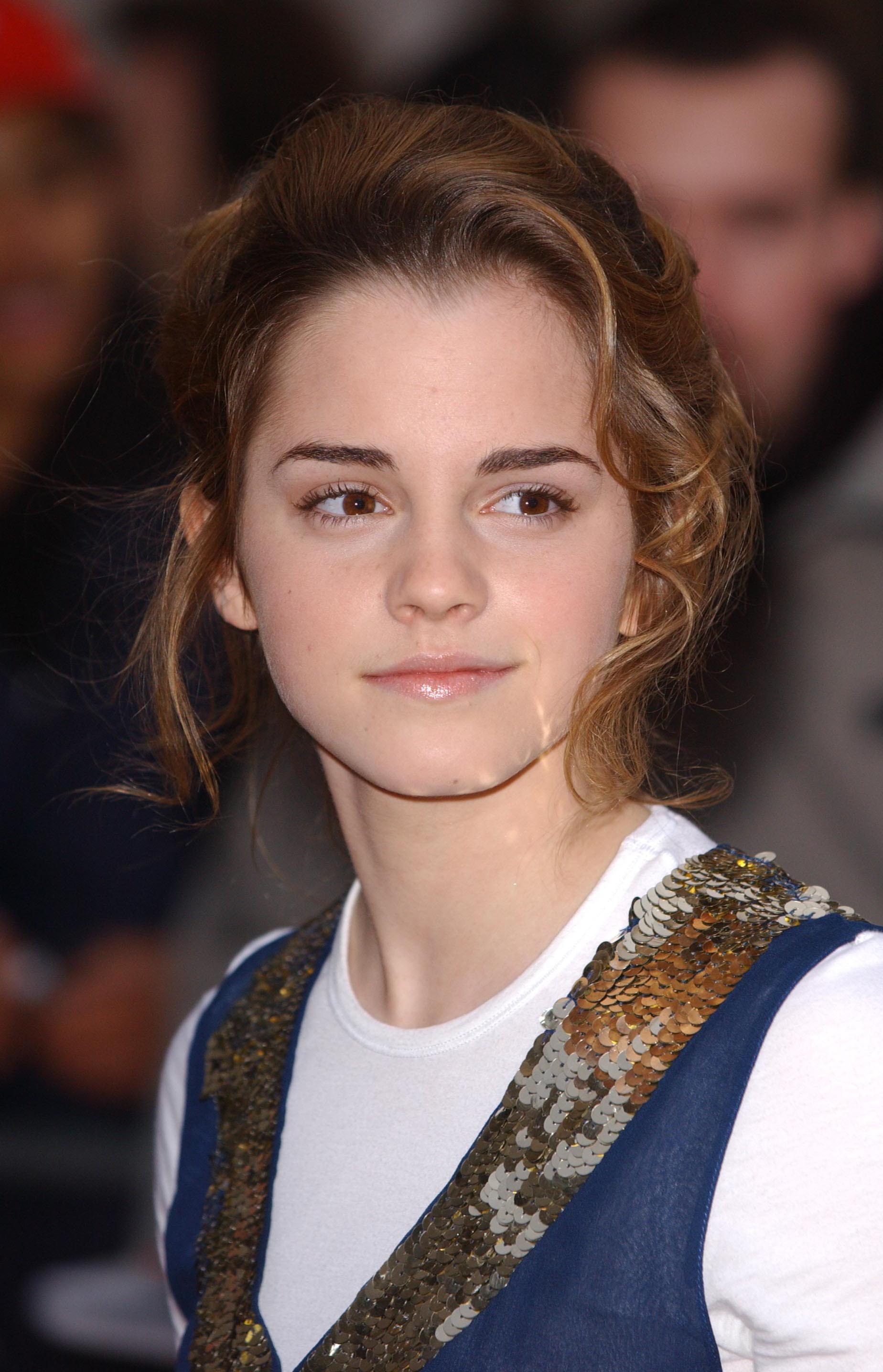This image is a detailed color photograph of the renowned actress Emma Watson, known for her role in the Harry Potter series during her younger years, likely around the fourth or fifth film. Emma is captured in the foreground with a backdrop that is blurred, rendering the few visible individuals indistinct. Her light brown hair is styled up in a bun, with soft curls and wisps framing her face. She has brown eyes, accentuated by mascara, and is wearing natural, light pink lip gloss which gives a shiny appearance. Emma dons a white shirt underneath a navy blue vest, which is adorned with reflective gold and silver sequins across the shoulders. Her gaze is directed off to the right, accompanied by a subtle smile, indicating she might be interacting with someone out of the frame. The lighting suggests the use of flash, highlighting her face against a softly illuminated background.